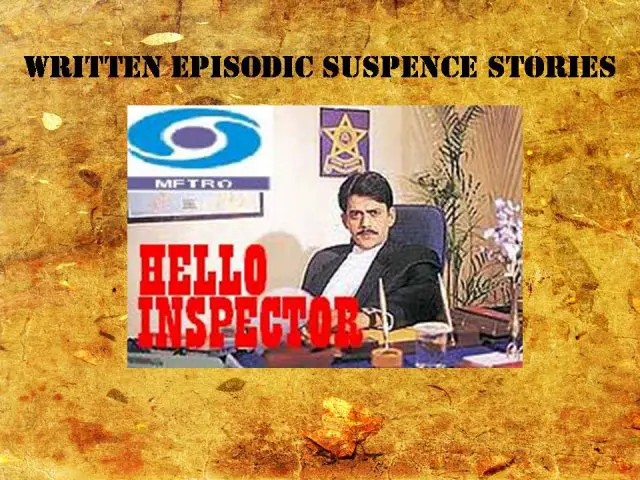In front of a textured brownstone background, an ad or slide prominently displays the text, "Written Episodic Suspense Stories" in bold black letters at the top. Below this headline, a serious-looking man, reminiscent of the actor from "Fear and Loathing in Las Vegas," is seated in a high-back blue office chair. He appears to be of mixed ethnicity with medium-length black hair and a black mustache, wearing a white dress shirt under a black coat. The office setting features a desk cluttered with various objects, including a vase with flowers and a glass. Behind him are tan walls adorned with a framed golden star and an emblem resembling a purple yin-yang with blue swirls encircling it. To the left of the man, the word "METRO" is inscribed, and the phrase "Hello Inspector" is boldly displayed in large red letters. The man stares directly at the camera, bringing a sense of gravity to the scene.